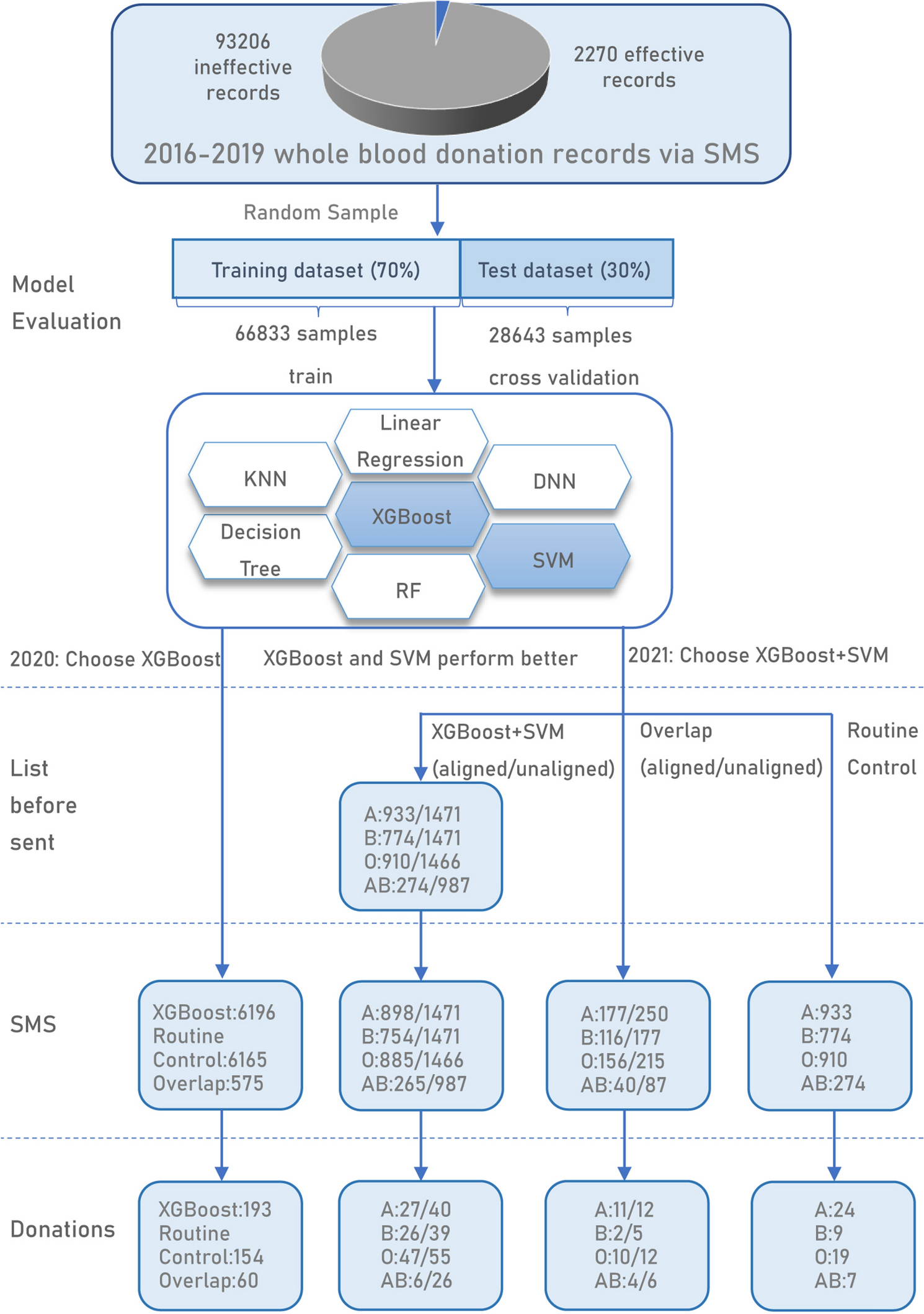The illustration showcases a detailed activity flowchart and data composition diagram on a white background, centered around the analysis of blood donation records via SMS from 2016 to 2019. At the top of the image, a focal heading reads "2016 to 2019 Whole Blood Donation Records via SMS." Directly below, a pie chart with grey and blue segments identifies 93,206 ineffective records on the left and 2,270 effective records on the right. 

Arrows lead downwards from the pie chart to indicate the division of data sets into a training data set of 70% and a test data set of 30%. This is followed by another section with geometric figures, including irregular hexagonal shapes and rectangles in white and blue colors. These geometric shapes contain further data, tables, numbers, and text, including references to analytical models such as linear regression, XG Boost, and Random Forest (RF).

Towards the bottom of the diagram, there are blue squares and additional information boxes labeled with different statistics, including a list comparing 'Before Sent SMS' with 'Donations'. The entire flowchart is rich in detail, exemplifying a meticulous layout of data analytics for blood donation records.